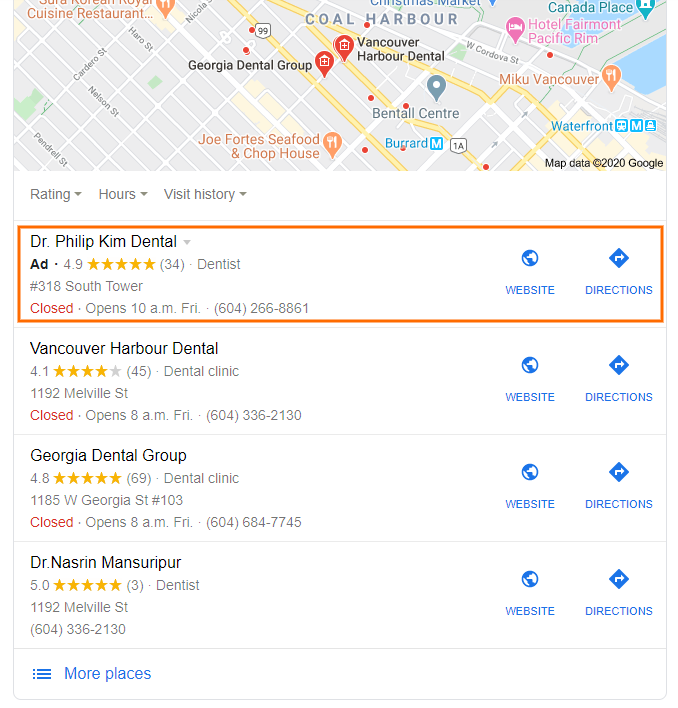The image displays a search results page for dentists, dominated by a wide, gray banner stretching from left to right at the top. This banner features a grid of white streets labeled with various company, restaurant, and dentist names in different colors. Below this, the page has a white background with a dark gray header containing clickable options for "Rating," "Hours," and "Visit History," which expand to reveal more information.

Underneath this header is an orange box spanning the page horizontally. Inside it, in black lettering, it reads "Dr. Philip Kim Dental," accompanied by the dentist’s rating, stars, and hours of operation. To the right of this information, there is a blue circular button labeled "Website" and a blue square button with an arrow labeled "Directions;" both are clickable for further details.

The layout repeats for three more dentists. The second entry is for "Vancouver Harbor Dental," with the same type of information and clickable options. The third is "Georgia Dental Group," followed by the fourth listing for "Dr. Nasrin Mansurapur." Each listing provides comprehensive details including ratings, hours, and contact information.

At the bottom of the page, additional navigation options are available in the form of blue lines and dots, with a clickable "More Places" link to explore further information about other dental offices.